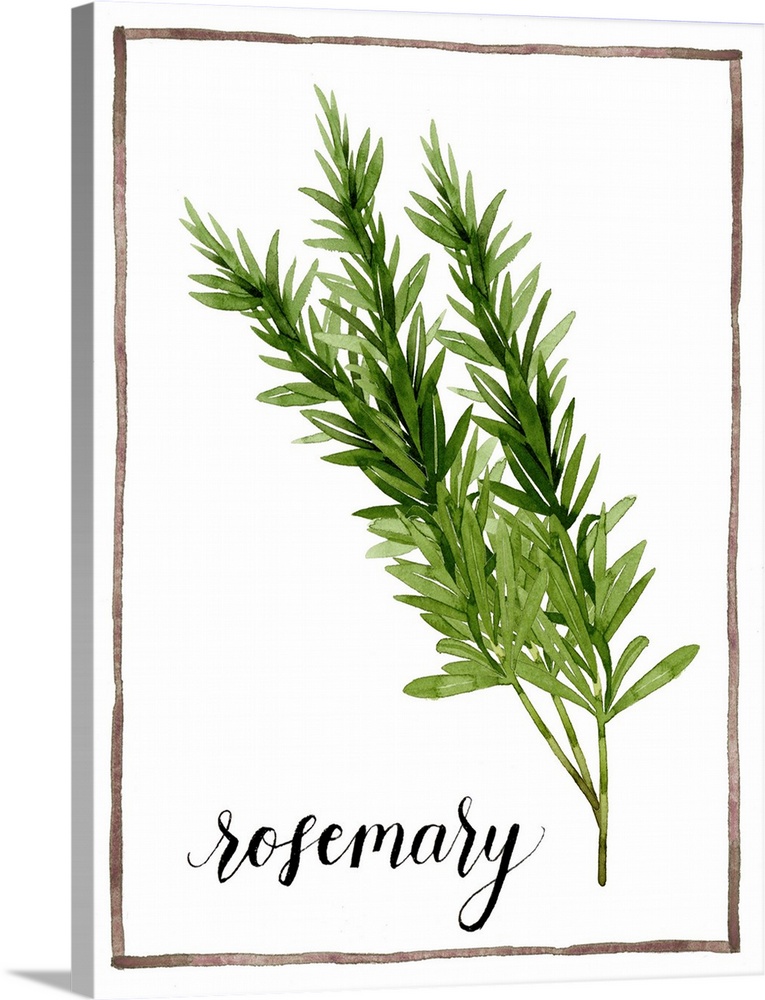This image is a detailed drawing on a canvas print featuring a vividly illustrated rosemary plant. The artwork depicts three tall stalks of rosemary emerging from a single stem, with varying shades of green, ranging from lighter hues to dark green accents. The leaves, resembling spikes, densely cover the entire stems from bottom to top, leaving no part of the stem visible. The background of the image is solid white, enhancing the clarity of the green herb. At the bottom of the canvas, "rosemary" is hand-scripted in elegant black cursive. Surrounding the artwork is a painted dark brown rectangular border, adding a refined touch to the piece. The sides of the canvas retain a white color, giving it a clean and polished appearance. The overall composition is crisp and sleek, showcasing a blend of textures and shades, making it both a visually striking and detailed representation of the rosemary plant.